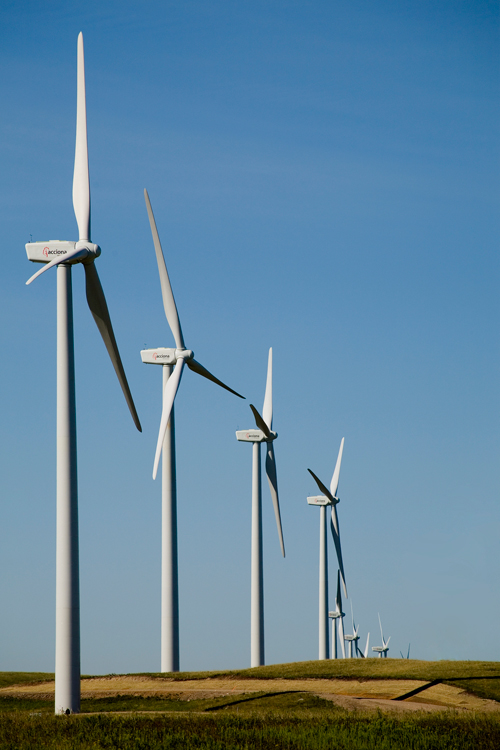This photograph captures a scenic outdoor setting during the daytime featuring a series of modern, white wind turbines. The image, taken from the viewpoint of someone standing and observing a row of turbines, presents seven to eight tall, metal structures with three large blades each. The turbines are aligned in a way that they appear to get progressively smaller as they stretch from left to right, creating an illusion of decreasing size. They stand on a well-maintained field with dark green grasses and patches of brown soil, reminiscent of a vast, open farm landscape. The sky above is a crisp, clear blue with no clouds in sight. At the top of each turbine, there is some text and possibly a logo in black and orange, though it's difficult to decipher. The detailed blades and towers look pristine and well-maintained, suggesting they are relatively new installations. The photograph exudes a picturesque and serene atmosphere, highlighting the blend of advanced technology and natural beauty.